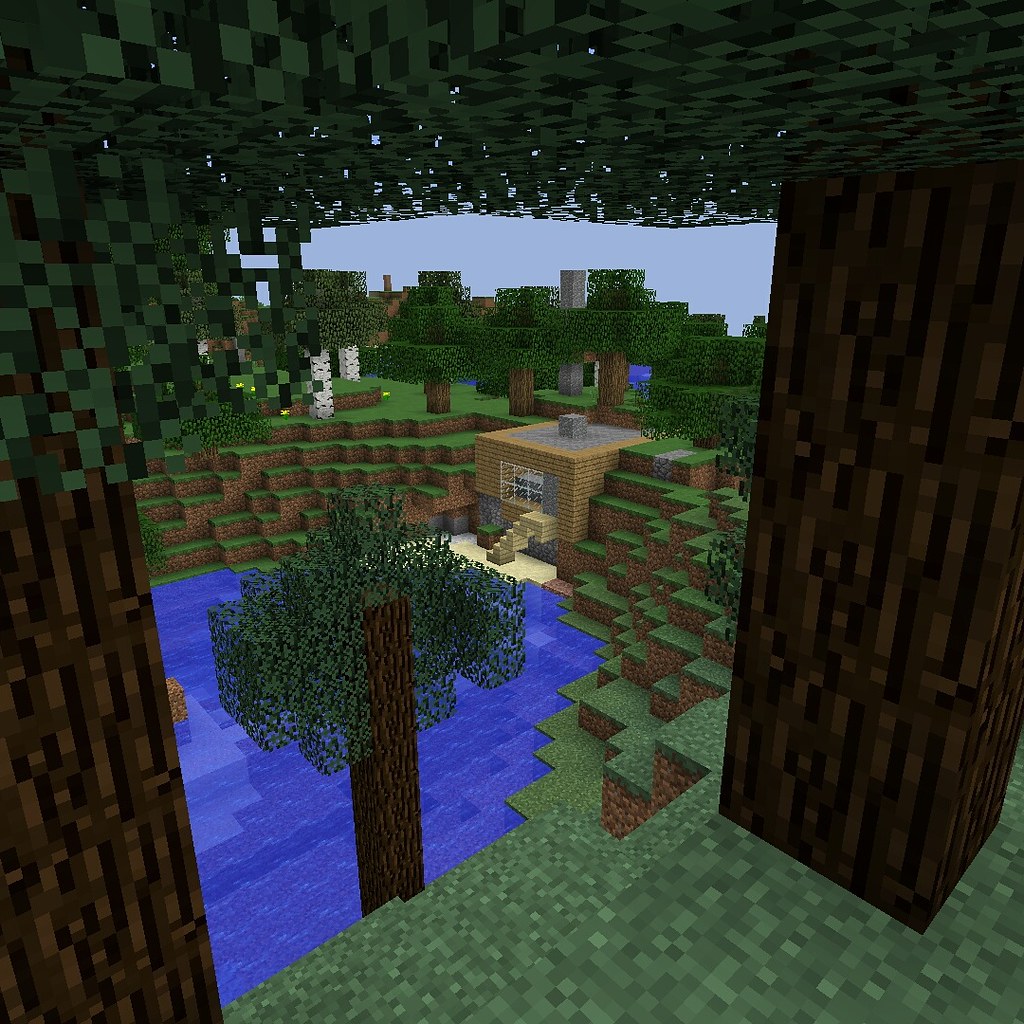This image appears to be from the popular game Minecraft. It showcases a serene landscape under a light blue sky, featuring a grove of trees and some scattered bushes adorned with purple flowers. Nestled into the side of a hill is a quaint house crafted from light brown materials. The front of the house is marked by six windows, and a tall staircase leads to the front door, which is surrounded by a dirt pathway. The house is positioned near the edge of a calm pond, adding to the picturesque setting. In the background, there are more hills and a few additional trees. The photo perspective is taken through the frame of two trees, positioned on the left and the right, with one more tree visible in the middle, partially submerged at the pond's edge.